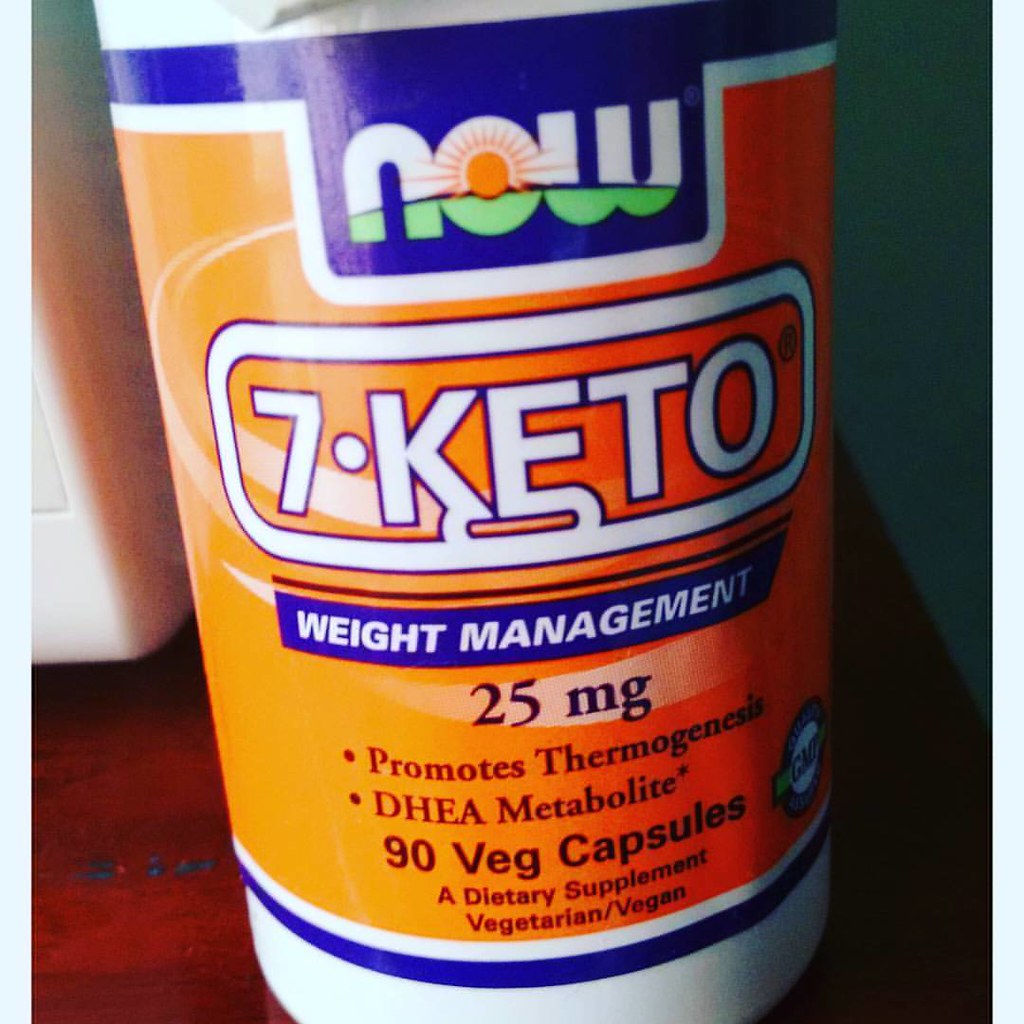This close-up photograph showcases a cylindrical supplement bottle predominantly orange in color, with dark blue and white sections at the top and bottom, respectively. The bottle is positioned on a maroon-brown countertop, next to the partial view of a white microwave, identifiable by the light gray edge of a button.

The bottle's label is detailed, starting at the top with bold blue text reading "now," where the "O" features an orange sun with extending rays. Each letter of "now" incorporates a dark blue curve with a green underside. Below this, in white text with a blue backdrop, it reads "7-KETO," followed by "weight management" on another blue background. Additional information includes "25 mg" in black text, and two bullet points: "promotes thermogenesis" and "DHEA metabolite." The label also mentions "90 veg capsules" and specifies it as "a dietary supplement" suitable for both vegetarians and vegans.

The background includes a blue section on the right side and a dark brown area at the bottom, alongside a logo indicating "GMO" inside a white circle with a blue border on the right side of the label.